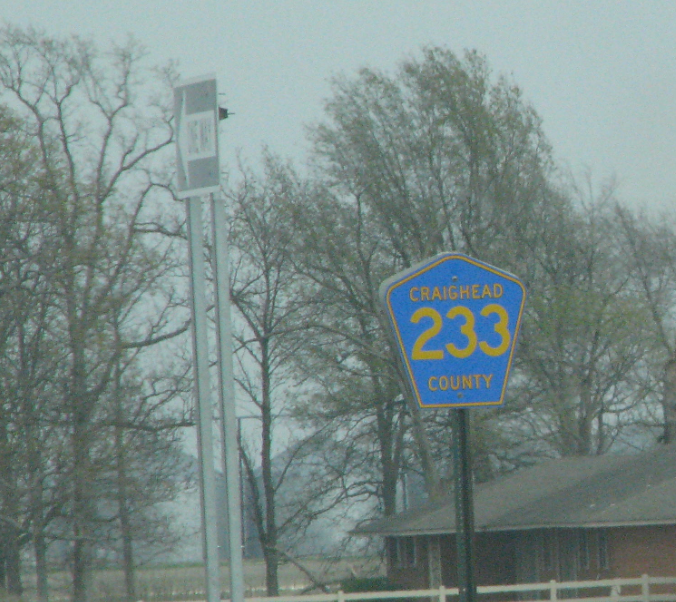A 1950s brick ranch house is situated by the side of a road, partially enclosed by a white rail fence. The scene has a faded appearance, neither sharp nor blurry. To the left center of the image stands a one-way street sign, and towards the right center, there's a metal pole with a blue, pointed-top street sign that reads "Craghead, 233 County" in yellow font. The background features an array of trees that appear to be either budding in early spring or still barren from winter. The sky is a muted blue-gray, adding to the nostalgic and subdued atmosphere of the scene.